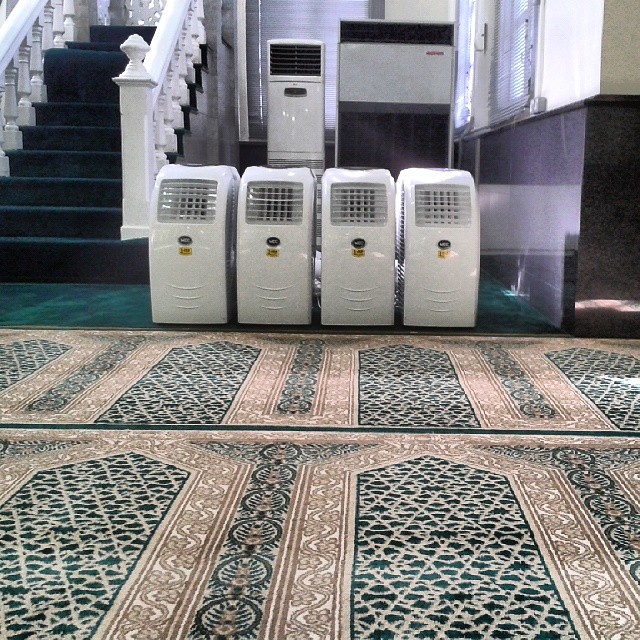This indoor digital photograph captures a scene with a black carpeted staircase featuring large white handrails on the left. Adjacent to the staircase are two mechanical devices: one smaller white device with a black square on top and another larger one composed of a black top, followed by a large silver rectangle, and a black base. The right side of the picture shows a wall that transitions from white at the top to a black marble finish at the bottom. In the foreground, there is a detailed tan carpet with intricate black designs, leading to a black carpet area similar to that of the stairs. On this black carpet, lined up side by side, are four white devices with gray slotted fronts and black logos with unreadable white text, beneath which are yellow triangles with black text. Behind these four machines, positioned towards the left, are two additional white and black devices that resemble the previously mentioned machines, possibly air conditioning units or heaters, one of which looks like an ice machine. The presence of blinds over windows suggests that the area may be a hallway in an old hotel.